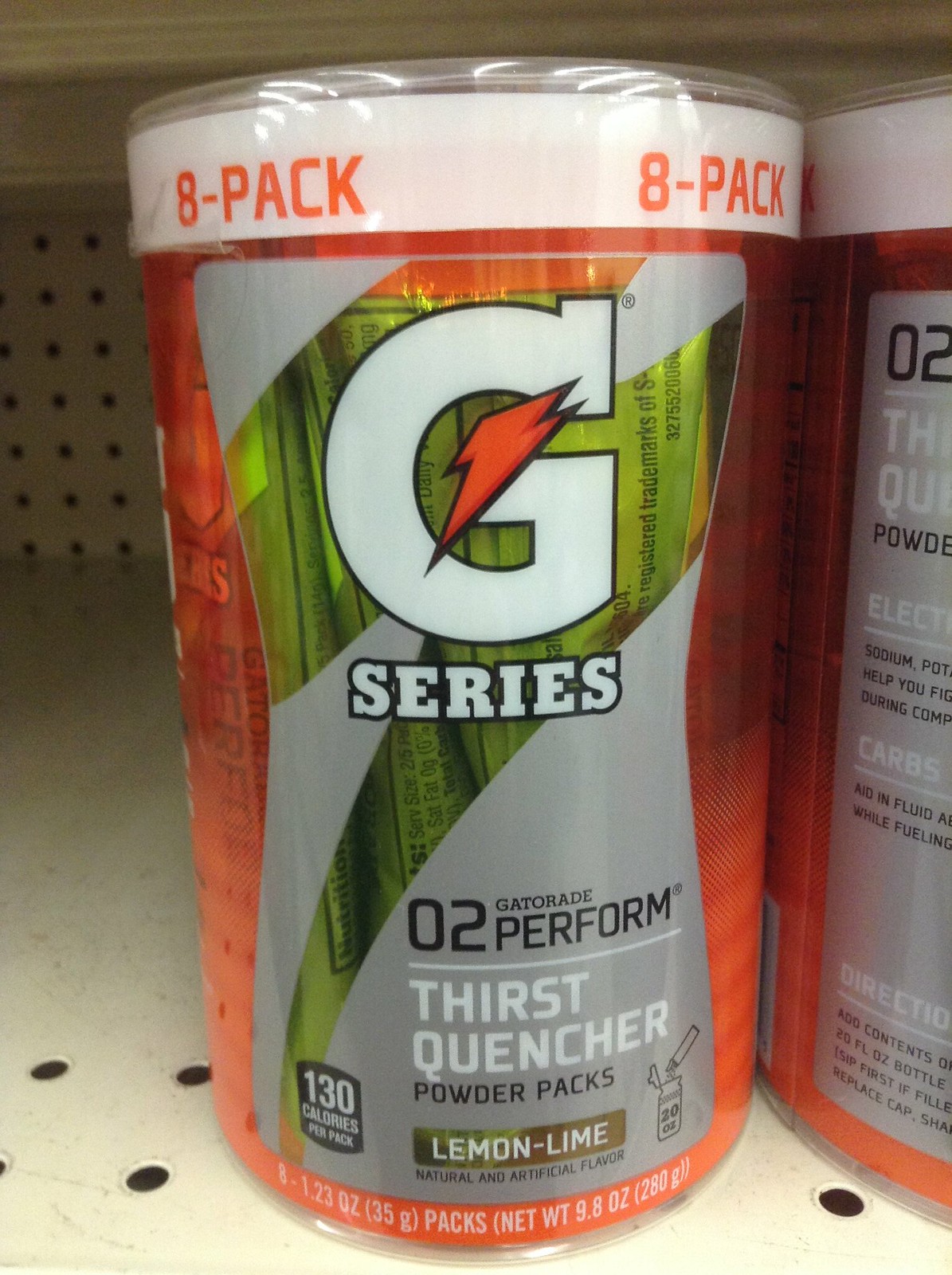This up-close photograph features a prominently displayed container of Gatorade powder packs against an off-white background. The product is centrally located on a metal shelf, with black perforated holes visible in the shelf itself. The container is tall and round, with a distinct packaging design.

At the top of the container, there is a clear plastic section followed by a white strip encircling it. The orange text on the white strip reads "8 pack." 

Dominating the center of the container is a gray label with a detailed design. A large capital letter "G," white and outlined in black, occupies the top center position. Inside the "G" is the iconic red Gatorade lightning bolt. Directly underneath, in capital white letters outlined in black, is the word "SERIES."

Two green strips intersect horizontally behind and below the "G." In the bottom right of the label, the black text reads "0 TO PERFORM," underlined by a white line. 

The text continues below in white letters with "THIRST QUENCHER," followed by "POWDER PACKS" in black. At the base of the label, a brown rectangle with white text reads "LEMON-LIME." The primary color of the container's background is a bold red, making the detailed label and text stand out prominently.